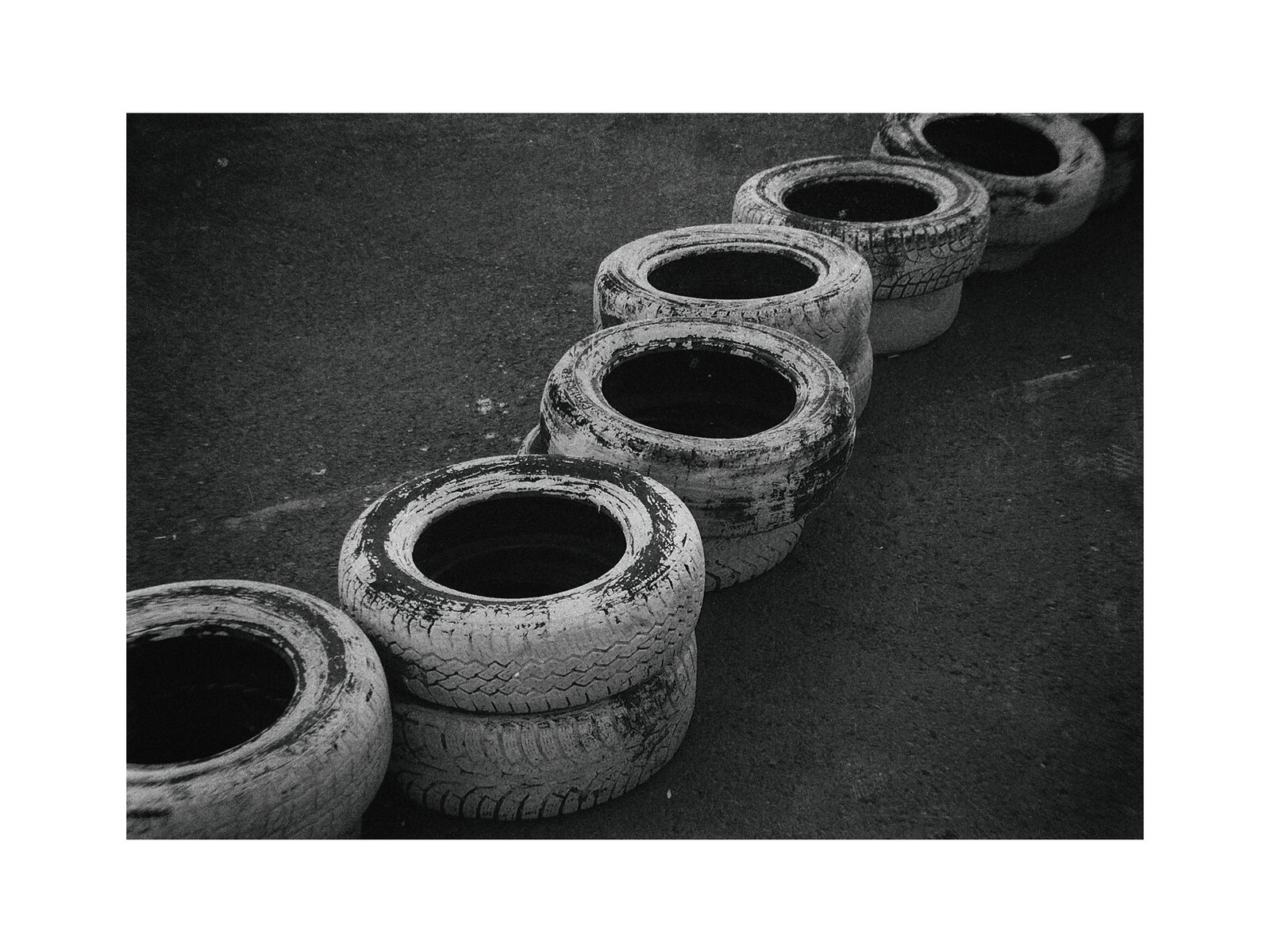The black and white photograph depicts a serpentine row of twelve tires, arranged in six stacks of two that appear to form a loose, wavy line on a black asphalt surface. These old tires, which show signs of wear and tear, are painted white with patches where the paint has rubbed off, revealing the black rubber beneath. The tires are neatly paired but give off a slightly disordered appearance, with the upper tires occasionally misaligned with those beneath them. Open at the top, the inner black of the tires is visible, and no plants or other objects are present within them. The scene appears muted, suggesting an overcast setting or the inherent nature of the black and white photography, possibly mimicking the edge of a go-kart track or some sort of makeshift barrier.